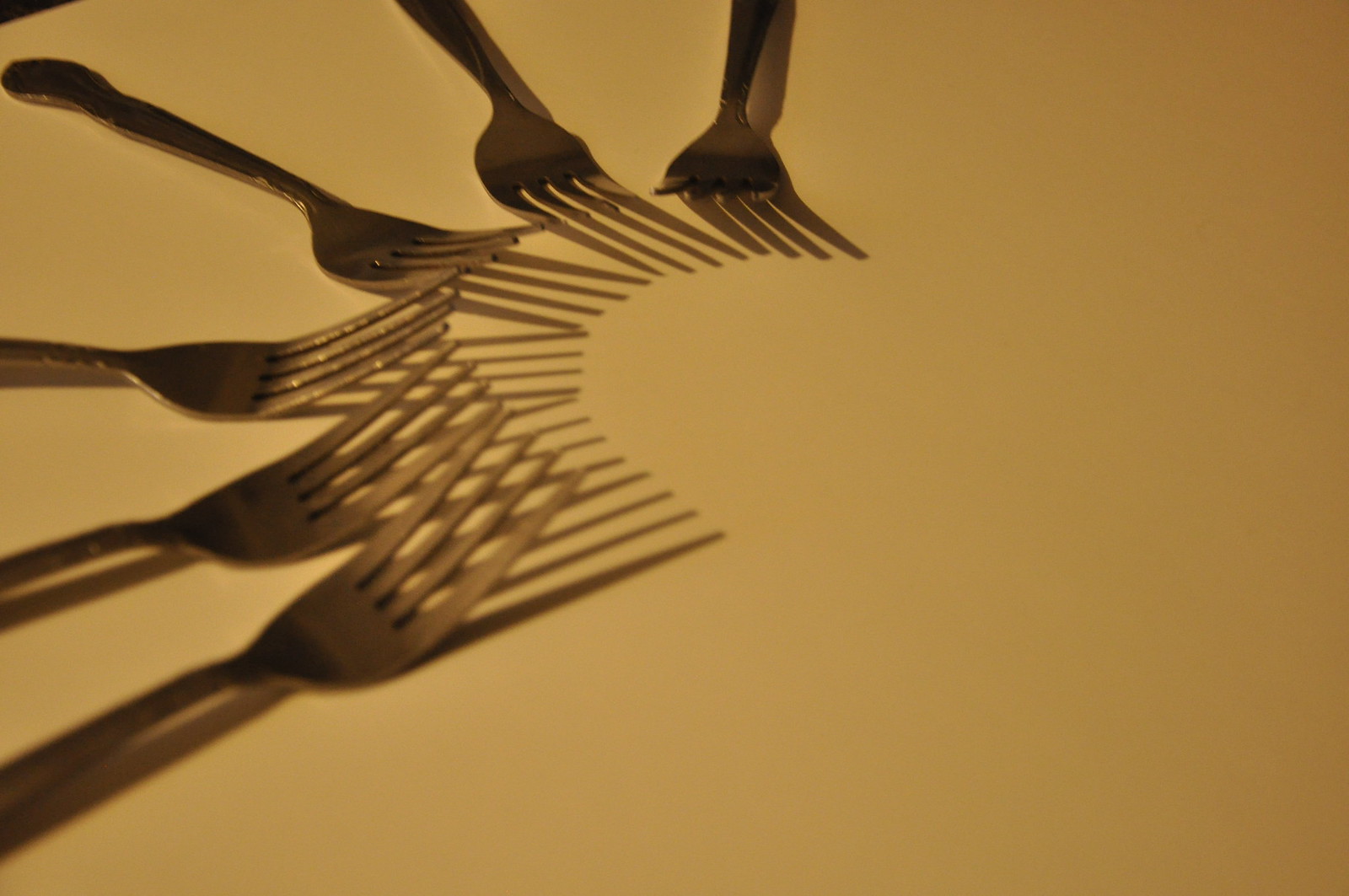This photograph captures six intricately designed silver forks, each with four slightly curved tines, arranged in a precise half-circle. They rest on a flat surface that appears off-white but is bathed in a golden yellow light, giving it a warm, beige tint. The forks' polished surfaces reflect this light, enhancing their metallic sheen. Positioned with their tips touching, the forks form a seamless arc, with no gaps between the points. The light source, coming from the upper left corner, casts distinct shadows of the tines beneath each fork, converging towards the center and reinforcing the semicircular composition. The handles of the forks are curvaceous and elaborate, adding to their elegance.